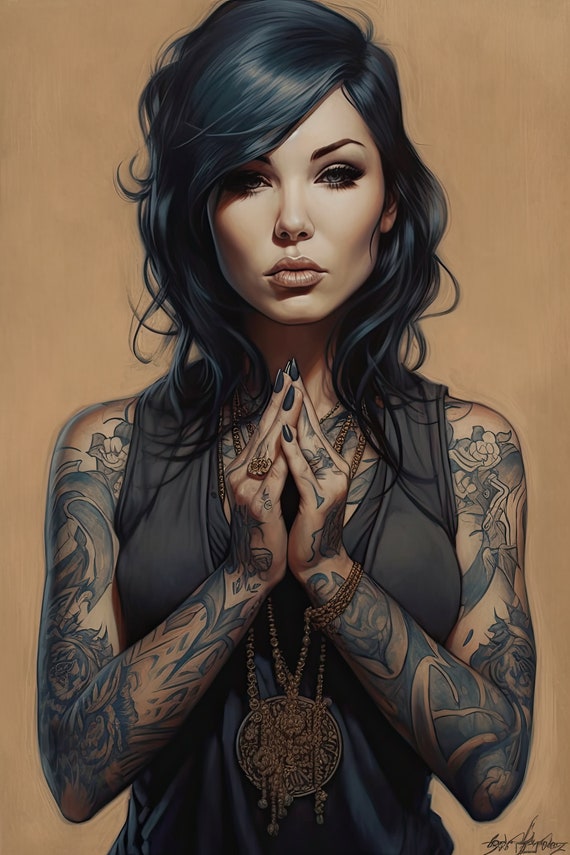The detailed, hand-rendered image, possibly illustrated in colored pencil or pastels, depicts a young brunette woman reminiscent of a very young Marie Osmond. Her long dark hair cascades to her shoulders, complementing her thick black eyelashes, arched eyebrows, and pouty mouth. She has a pale complexion and intense, heavy makeup that accentuates her dark eyes. She wears a black sleeveless top that reveals her extensive tattoo sleeves, stretching from her shoulders down to her hands. The tattoos continue onto her upper chest, adding to the elaborate design. Her hands are clasped together just below her chest in a gesture that suggests a prayer-like pose, adorned with black fingernail polish and a ring on her right ring finger. Around her neck, she dons heavy gold medallion necklaces with large pendants that hang down over her torso. The image, against a light beige or brown background, is signed by the artist in the bottom right corner, framing her striking presence and detailed tattoos.